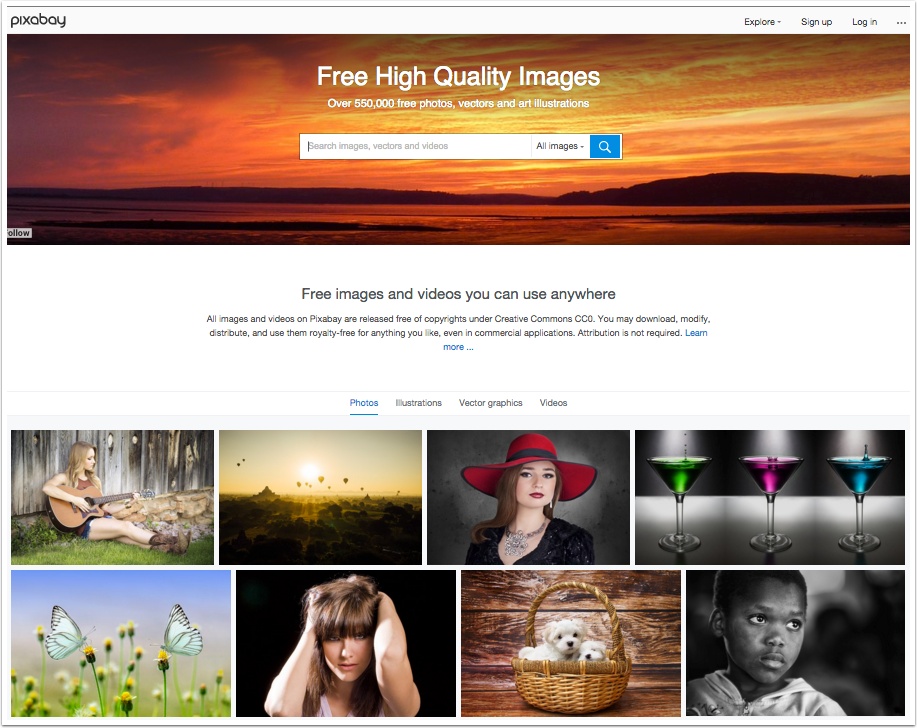The image is a screenshot of the Pixabay website. At the top left corner, the site's logo "Pixabay" is prominently displayed. On the upper right-hand corner, navigation options including "Explore," "Sign Up," and "Log In" are clearly visible. 

The main section of the website features a visually stunning image of a sunset, where the sky is painted in beautiful shades of orange, yellow, and rich dark red. The silhouette of mountains is outlined against this vibrant backdrop. Overlaying the sunset image, text announces, "Free high-quality images: over 555,000 free photos, vectors, and art illustrations."

Directly below this, a search bar is provided for users to explore the platform’s content. The next section highlights the website's offering with the statement, "Free images and videos you can use anywhere." It emphasizes that all images and videos on Pixabay are released free of copyright under Creative Commons CCO, allowing users to download, modify, distribute, or use them royalty-free for any purpose, including commercial applications. The note specifies that attribution is not required, and a "Learn more" link, highlighted in blue, is available for further information.

Beneath this section, categories such as "Photos," "Illustrations," "Vector Graphics," and "Videos" are listed. Displayed images in these categories include a variety of subjects: a girl playing guitar, a woman in a red hat, a basket filled with white puppies, a girl with brown hair holding her hands to her head, a young boy gazing into the distance, three wine glasses in green, pink, purple hues, butterflies resting on flower buds, and a picturesque sunset with birds flying in formation.